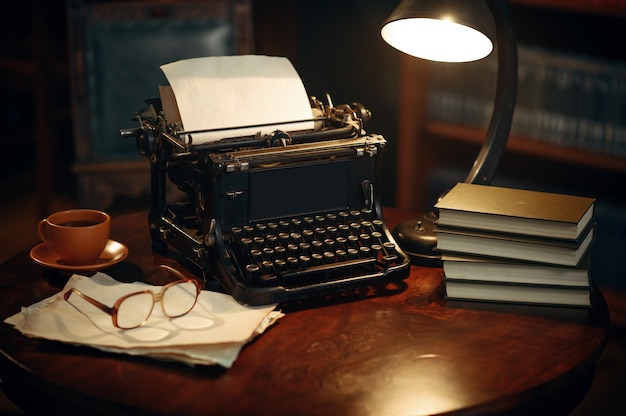The photograph captures an evocative, vintage workspace set on a dark, richly colored wooden table, perhaps mahogany or cherry wood. The centerpiece is an old, classic mechanical typewriter, featuring large, protruding keys and a body that cradles a sheet of paper. Positioned to the right of the typewriter is a sleek, curved black desk lamp emitting a warm white glow, illuminating the scene. Just beneath the lamp, a neat stack of four books suggests a scholarly atmosphere. To the left of the typewriter, a set of crinkled papers is topped with a pair of brown, round glasses.

Further back, a small coffee cup filled with dark, almost black coffee rests on a brown porcelain bowl, adding a lived-in feel to the workspace. In the background on the right, shelving can be faintly discerned, and to the left, there appears to be a blurry black leather chair with a wooden frame, contributing to the room's timeless ambiance. The overall setting exudes a sense of quiet, studious solitude, bathed in the lamp's light amidst an otherwise shadowy room.